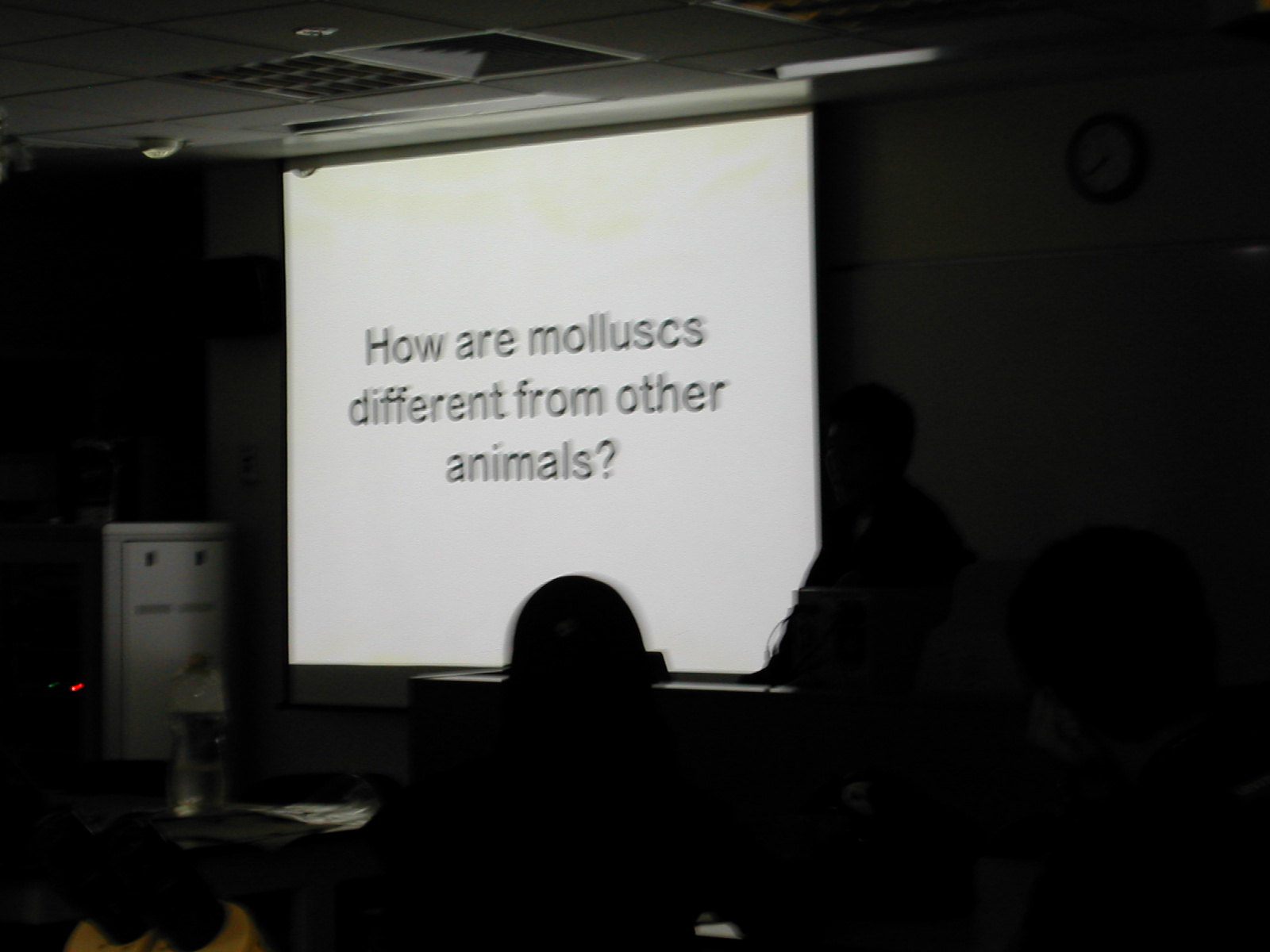This photograph captures a dark classroom where a presentation is taking place. The focal point is a projection screen at the front displaying a slide with the black text: "how are molluscs different from other animals?" centered on a white background. The room is predominantly dark, with just enough light from the screen to make out some details. The ceiling, partially visible, is mostly white with a vent. To the left of the screen stands a white cabinet, and below it, a desk with a water bottle can be seen. Partially obscuring the bottom of the projector is an ambiguous object, possibly a chair. On the right side of the screen, the faint outline of a person, possibly wearing glasses, is noticeable. At the lower right-hand corner of the image, the back of another person's head can be seen, seemingly resting on their hand. Despite the darkness, the atmosphere suggests an ongoing educational session focused on molluscs.